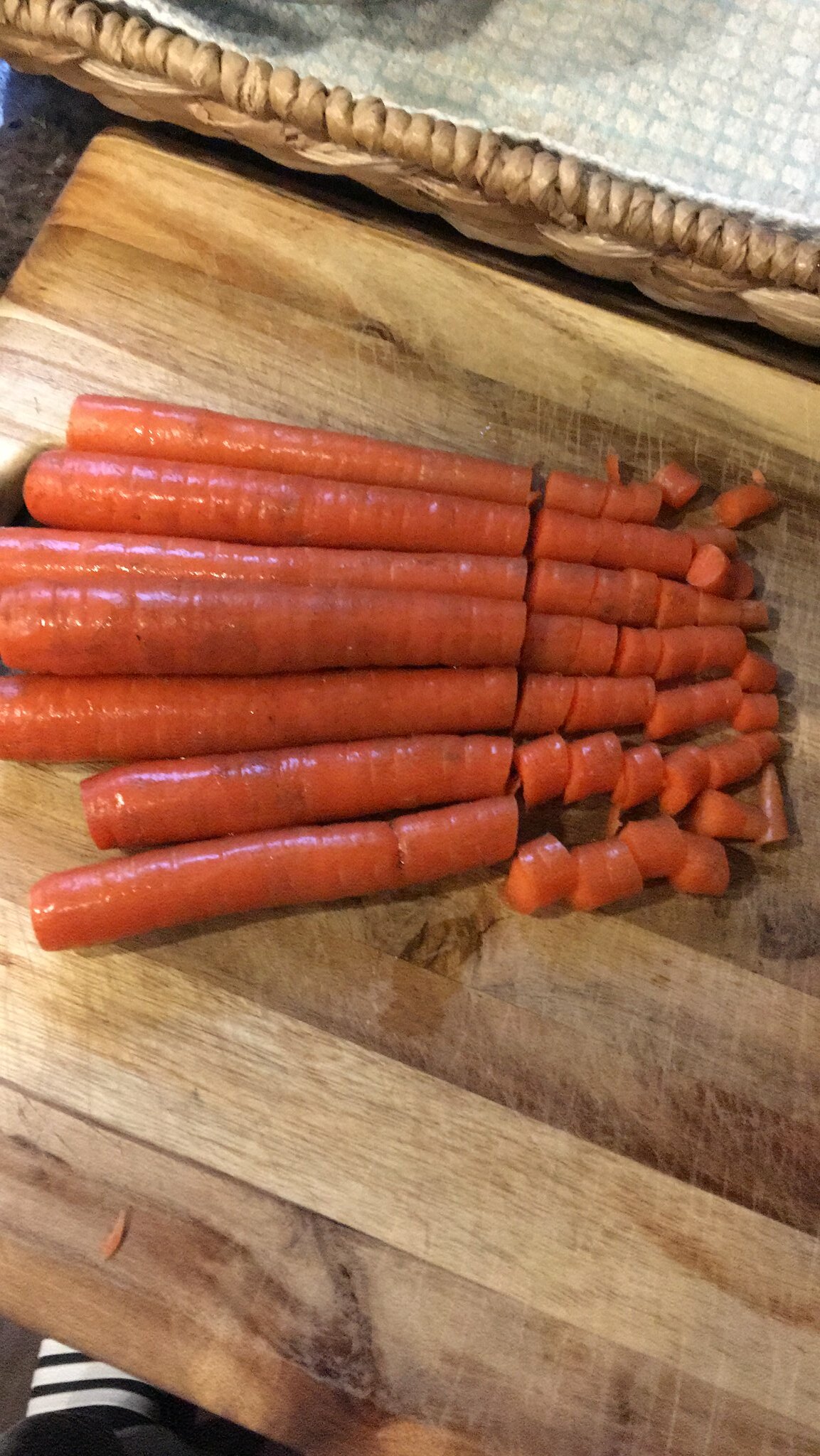In a cozy kitchen setting, a wooden cutting board rests on a dark granite countertop, adorned with seven perfectly lined-up, freshly rinsed carrots, boasting a shiny sheen. The bottom halves of the carrots have been meticulously chopped into small pieces, while the upper halves remain intact. A glimpse of a white and black striped sandal peeks into the bottom left corner of the image. Additionally, a woven wooden basket intrudes slightly into the foreground, adding a rustic charm to the scene.